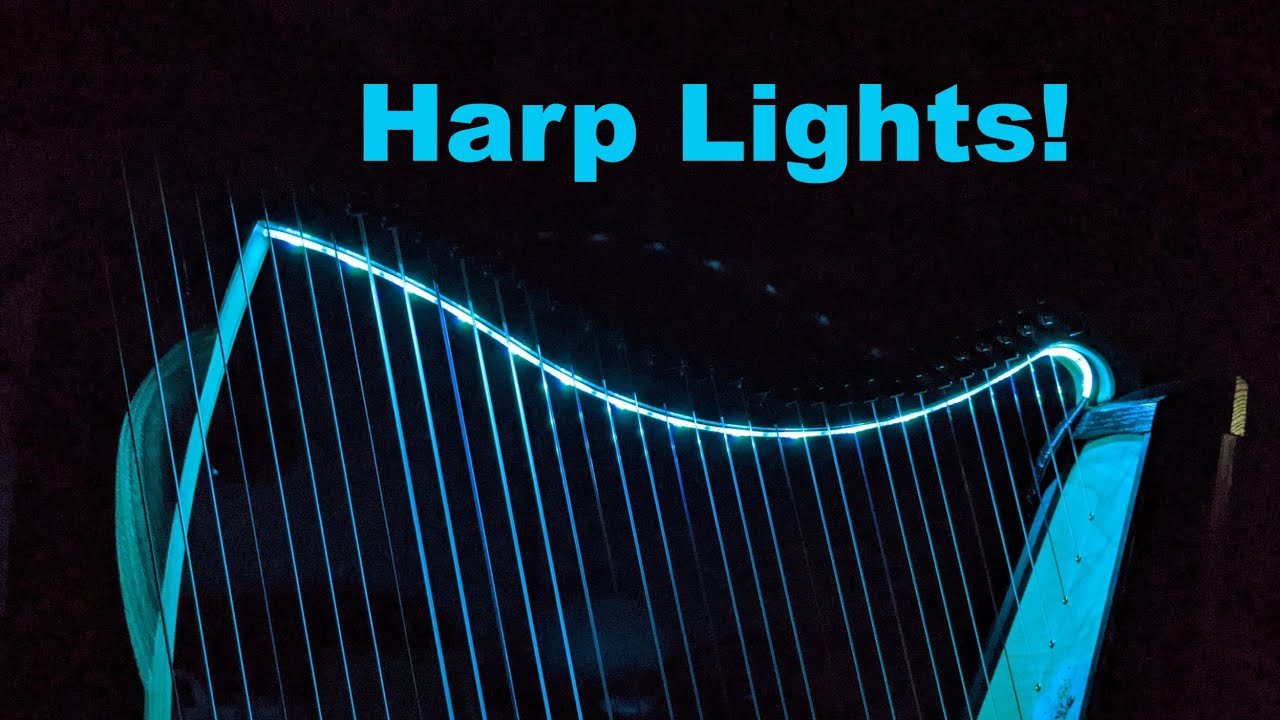In the photograph, a harp is prominently featured, illuminated by neon blue LED lights against a pitch-dark background. The top of the image has blue text that reads "HARP LIGHTS!" The harp itself is centrally positioned, with its strings visible and glowing due to the blue lights. The strings descend vertically through the dark surroundings, where the blue illumination accentuates them, creating a striking contrast. The LED strip runs along the top and inside edges of the harp, giving it a bright blue hue and causing parts of it to stand out sharply against the void-like backdrop. The background remains largely indiscernible, with some strings fading into the darkness where the light doesn't reach, giving the instrument an ethereal, almost ghostly appearance.